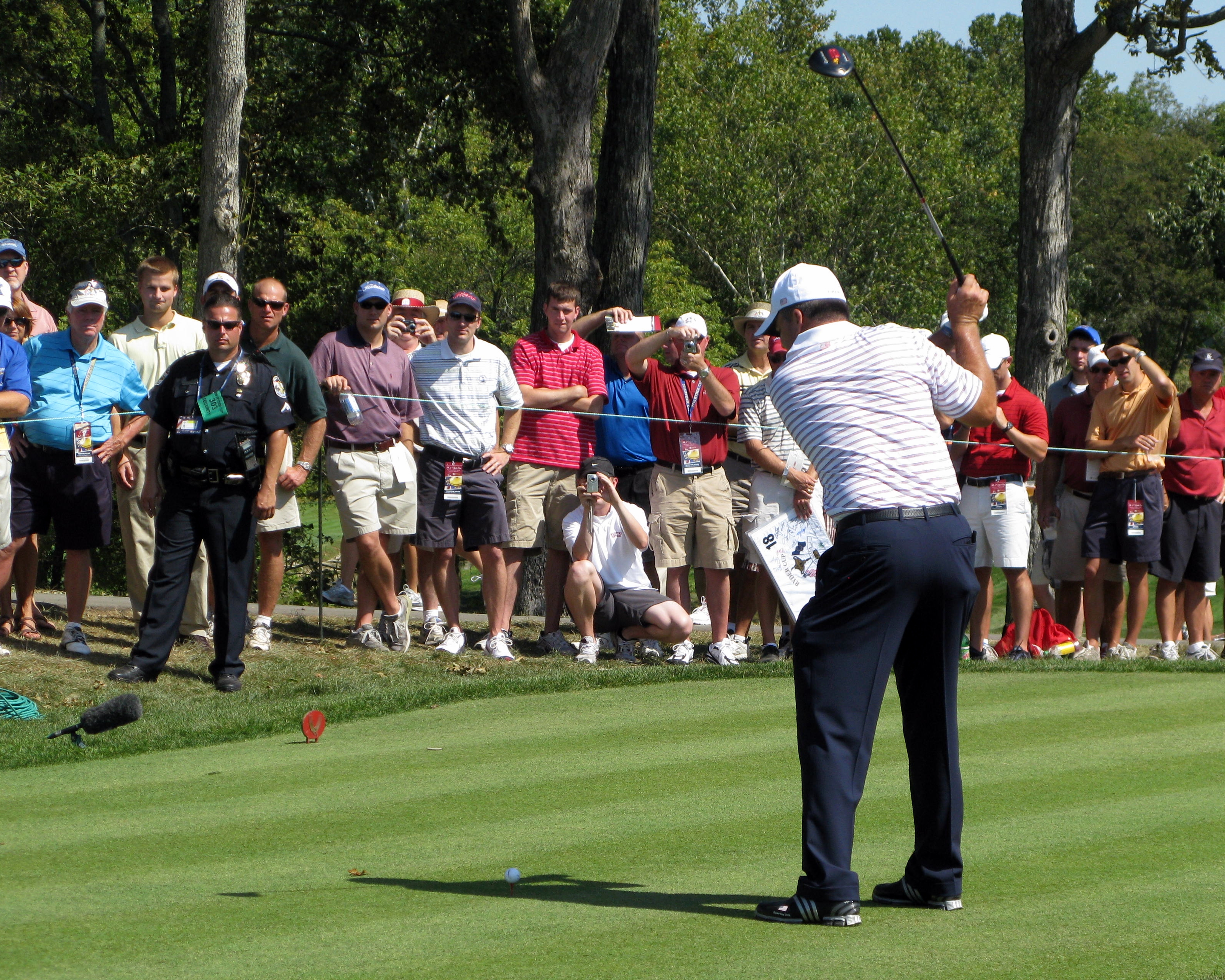In this outdoor photograph, a golfer, possibly resembling Tiger Woods but not clearly identifiable, is captured mid-swing with his back facing the camera. He is dressed in blue slacks that mimic a suit's appearance, a white cap, an Apollo shirt boasting black, white, and light blue stripes, and black Adidas shoes. His golf club is fully cocked backward, poised for a powerful swing. The golf ball is positioned on the grass, nestled within his shadow. The grass on the course displays a distinct pattern of dark and light green stripes, bordered by short bushes. To the left of the scene, a police officer stands vigilantly by the rope barrier, ensuring crowd control as numerous spectators, dressed in summery attire of shorts and short sleeves, watch the golfer intently. In the background, a lush array of trees and a glimpse of blue sky add depth to the image, with one tree humorously appearing to sprout from the officer's head.